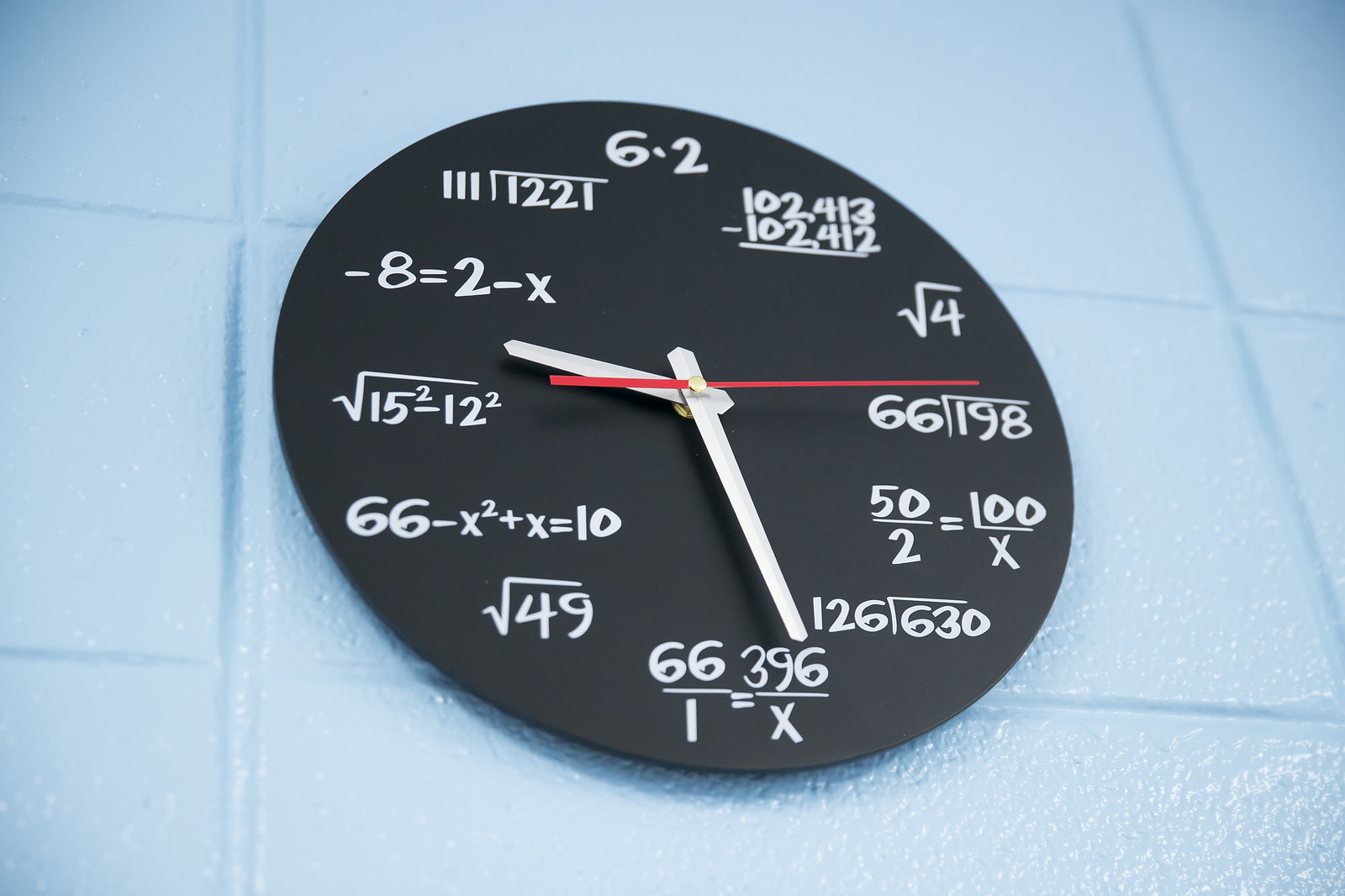This photo captures a uniquely designed clock mounted on a white-painted brick wall composed of large cement breeze blocks. The brick pattern is unusual, as the blocks are stacked directly on top of each other, creating a visually striking but structurally improbable arrangement. The image is taken from a low angle, with the photographer positioned slightly to the left, causing the clock face to tilt such that the number 12 leans towards the top left corner and the number 6 towards the bottom right.

The clock itself features a minimalist black face, with white hour and minute hands and a striking bright red second hand. What sets this clock apart is its creative use of mathematical formulas in place of traditional numerals. For instance, the 12 is represented by the formula "6 x 2," while the 2 is depicted as the square root of 4. Each number on the clock is cleverly substituted with a mathematical expression, making it an intriguing piece for anyone with a penchant for mathematics.